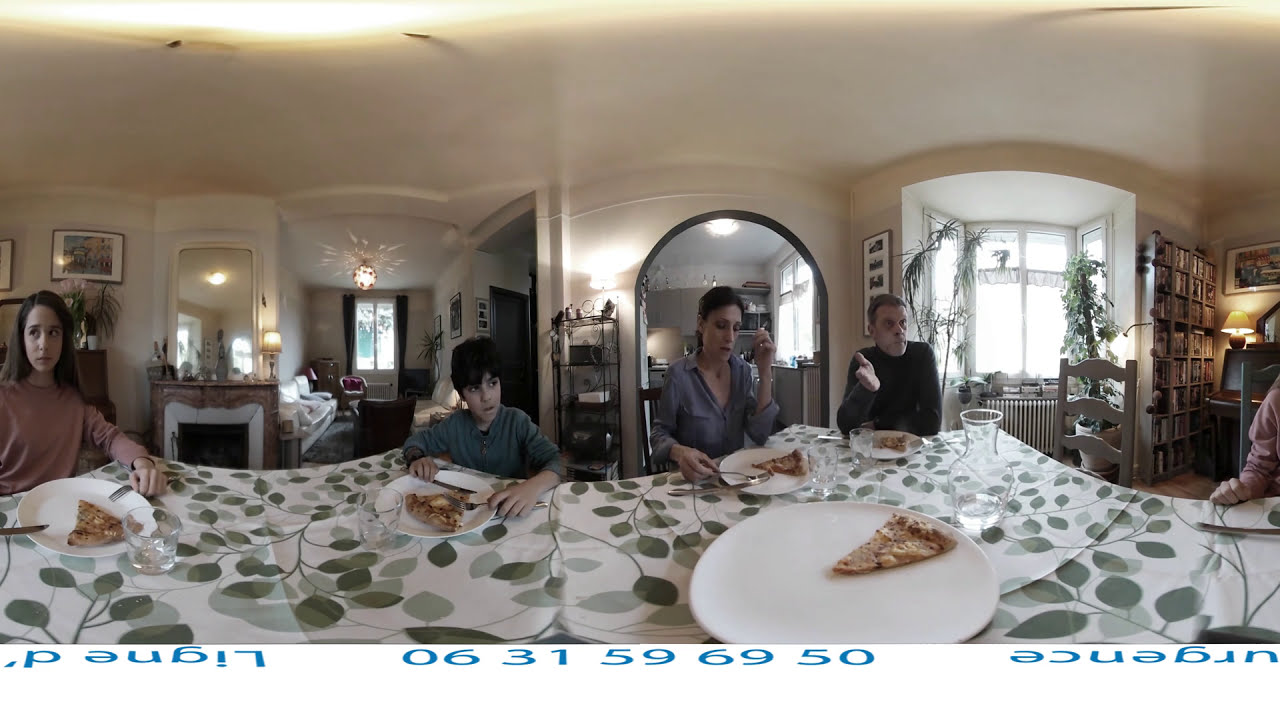The color photograph captures a warm family gathering of four people seated at a dining room table, enjoying slices of pizza. The table is adorned with a white tablecloth featuring a pattern of green leaves, adding a touch of nature. At the center of the table, there's a large round plate with a single slice of pizza remaining, while each person has their own smaller round white plate with a slice.

On the right side of the table, a man wearing a long-sleeved black shirt is actively gesturing with his hand, as if deep in conversation. Next to him, a woman in a gray v-neck long-sleeved shirt has her hand resting on her plate. Next to her is a young boy in a long-sleeved green shirt, who appears distracted, looking off to the right. Sitting on the left, a girl wearing a long-sleeved pink shirt is focused on her meal, her hands poised with a fork and knife.

The room's background details include an archway leading to a sunlit window, a hallway to the left, and a bookcase on the far right. The walls are adorned with a few pictures, and the ceiling is white, complementing the overall bright and cozy atmosphere of the dining area.